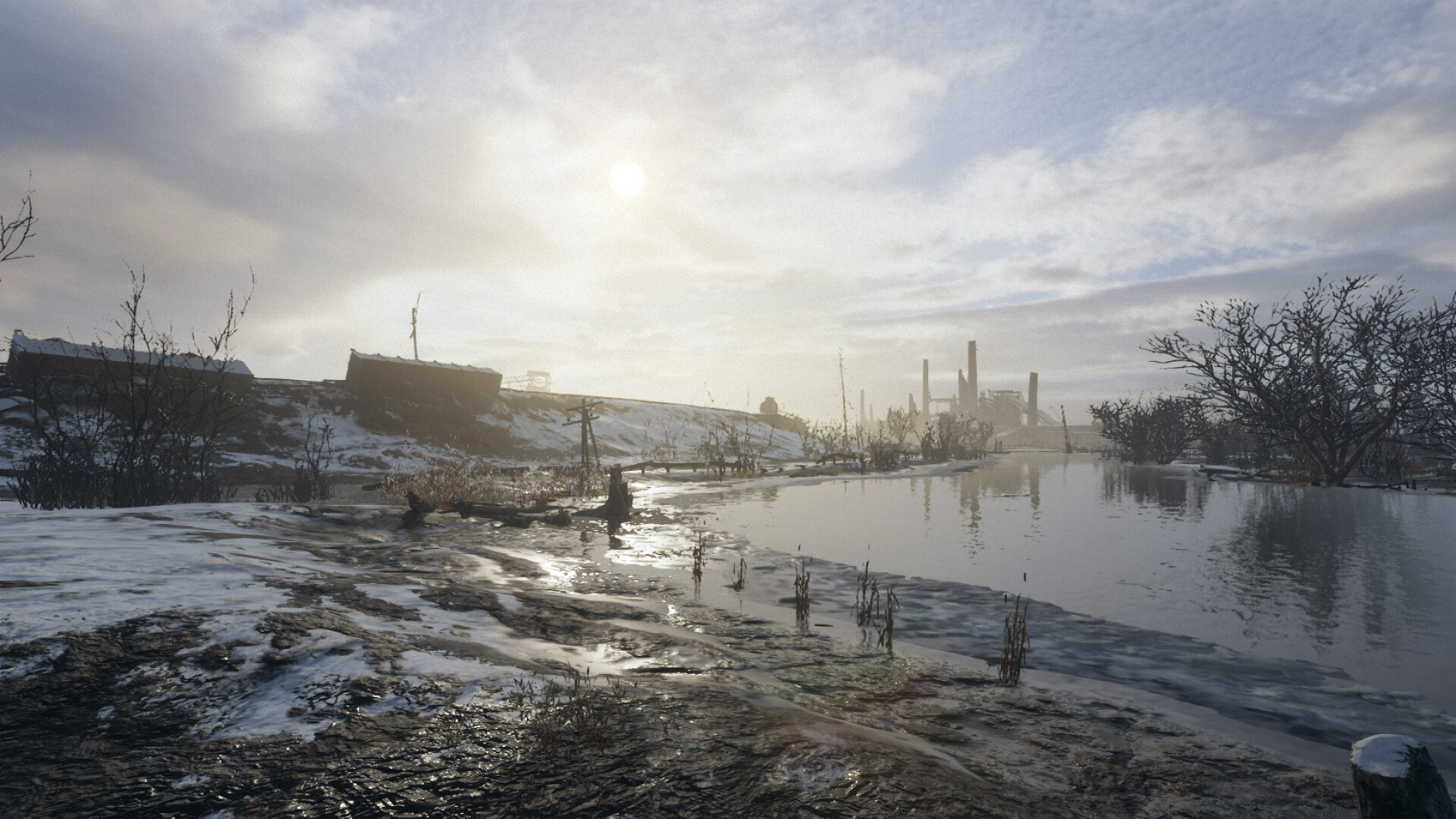In this winter scene, the landscape features a variety of elements. At the bottom foreground, there is a rocky terrain in shades of gray and brown, interspersed with patches of snow. To the left, snow predominantly covers the ground, creating a stark white contrast against the rocky background. On the right, a body of water reflects the sky, giving it a light grayish-blue hue. A leafless tree stands on the right edge, its image mirrored in the water below. On the left side of the scene, two dark brown rectangular structures are visible, adding a hint of human presence. In the background, several slender, vertical rod-shaped towers rise into the distance. The sky above is mostly white with clouds, punctuated by hints of blue and gray, particularly on the left side, suggesting a cold, tranquil winter day.